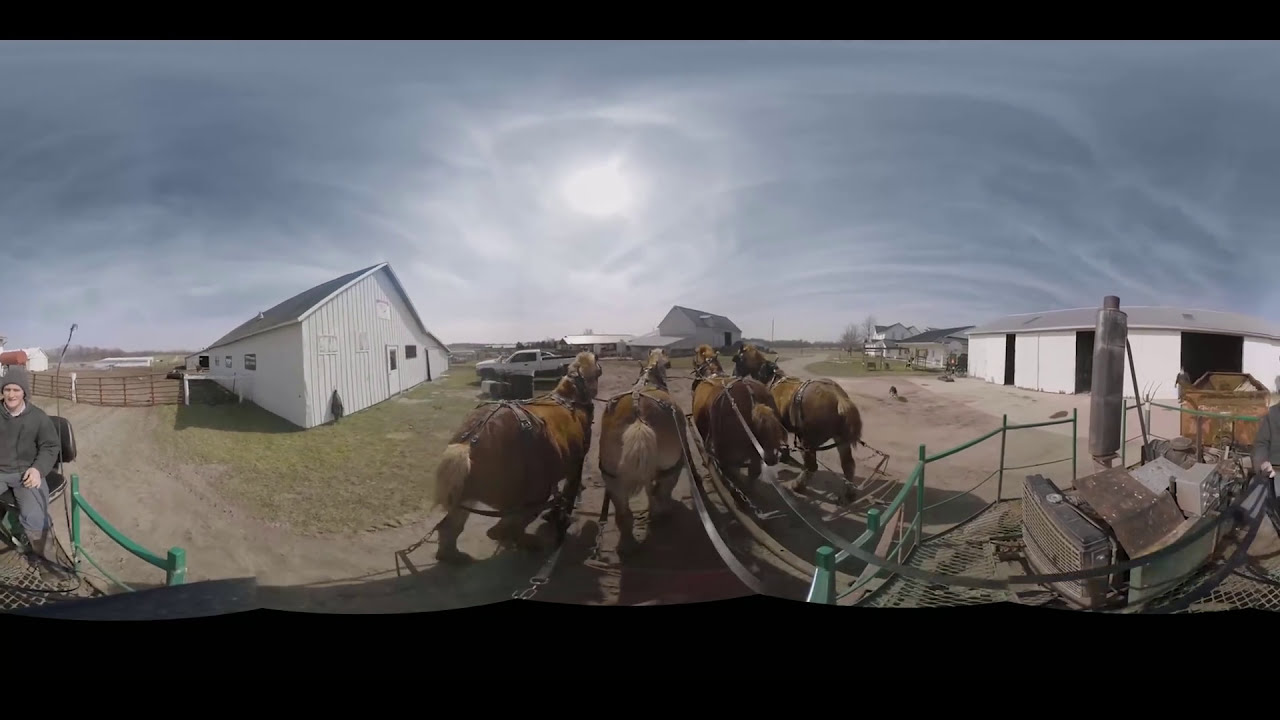In this richly detailed 360-degree photograph, a scene unfolds on a vintage farm that evokes a nostalgic, Western atmosphere. Dominating the center are four brown horses with short, cropped, lighter-colored tails, harnessed to large, green, mechanical farming equipment. They stand on a dirt road, epitomizing rural labor. Behind them, the expansive farmland sprawls with multiple white barn-style buildings and sheds. A white pickup truck is also visible, contributing to the authenticity of the pastoral setting. Scattered across the scene are several people and a few dogs, reinforcing the farm's bustling activity.

The photograph, taken during a dreary daytime, features an overcast sky with the sun peeking through thick, grayish-blue clouds, providing an almost ethereal lighting effect. This is accentuated by a Photoshop filter that gives the image a slightly edited, vintage touch. The person capturing this moment appears twice in the image due to the 360-degree camera setup. This individual is a young Caucasian man, dressed entirely in gray, from his skull cap to his long-sleeved shirt and pants. He is seated in a chair, seamlessly integrated into this panoramic view, which further illustrates the grandeur and tranquil disarray of everyday farm life. The photograph is framed with a narrow black header and a slightly larger footer, encapsulating this serene yet industrious rural panorama.